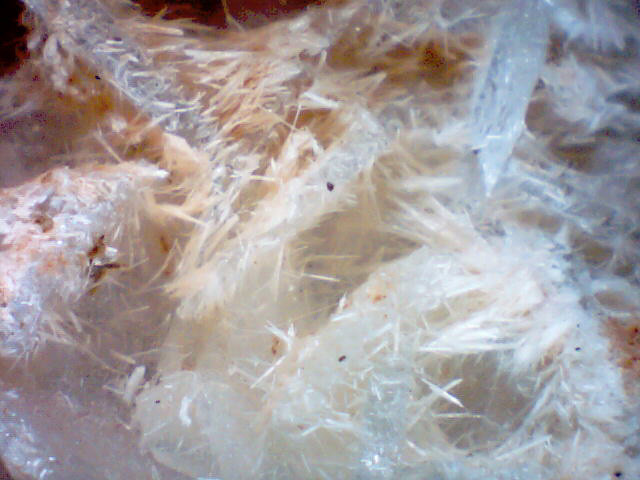This image is a close-up featuring delicate, flaky structures that resemble feathers with an array of varying colors. In the top left corner, a black background contrasts with intricate white and brownish strips, creating a striking visual effect. The left side of the image showcases a prominent white piece extending outward, while the middle and bottom sections feature scattered white areas. Towards the upper right-hand corner, wispy whitish feathers appear against a bluish backdrop, punctuated by a small brown area in the lower right-hand corner. The feathers themselves are composed of very fine, hair-like strands that radiate in multiple directions, with some forming cross or star-like patterns. The texture of the image hints at the fine and delicate consistency of the material, appearing almost like ice crystals or thin slivers of an unknown flaky substance, potentially resting on a surface akin to animal skin.